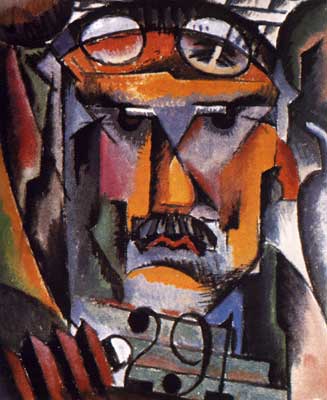This abstract painting features a vaguely humanoid face constructed from a chaotic yet deliberate jumble of geometric shapes and vibrant colors. Notable elements include triangular eyes and an orange, triangular nose, set against a kaleidoscope of blocky oranges, reds, grays, blues, blacks, a hint of green, and traces of yellow. The face is defined by striking red lips shaped like an 'M' and a distinguished gray, multi-toned mustache. Atop the head, shapes resembling glasses or goggles with two reflective ovals add an extra layer of intrigue. Surrounding the face, various geometric forms contribute to the painting’s dynamic composition. The lower section features the number "291" positioned on gray stairs that tilt to the right, accompanied by red stairs that appear almost upside-down or sideways. In the lower left, there's an enigmatic shape that could be interpreted as a plunger or part of an accordion, adding to the abstract mystery of the piece.